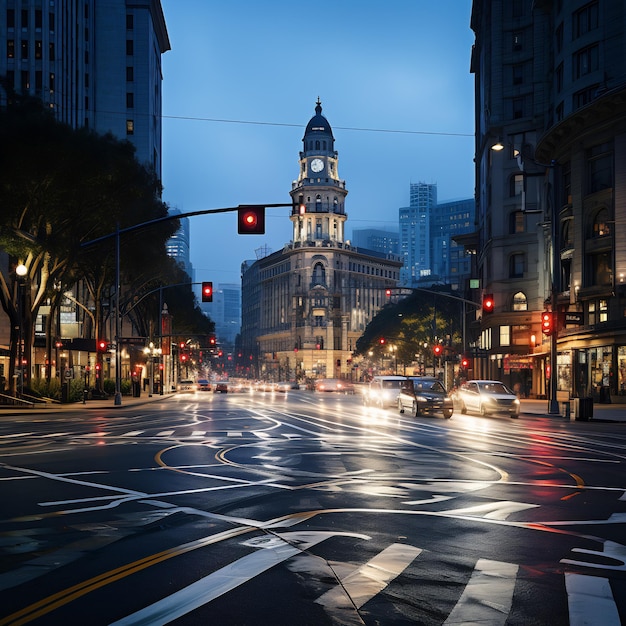This image, seemingly AI-generated, depicts a confusing nighttime intersection in the downtown district of a modern city. Taken from the vantage point in the middle of a crosswalk, the scene is illuminated by numerous streetlights and headlights reflecting off the asphalt. The intersection itself features a perplexing array of street lines, curves, and crosswalks, with some red dots and streetlights appearing oddly placed. Dominating the background is an older, triangular-shaped building with a clock tower and spire, evoking a European architectural style. Surrounding this focal point are high-rise apartment complexes and various shops, with a few people visible on the sidewalks, emphasizing the bustling, urban environment.